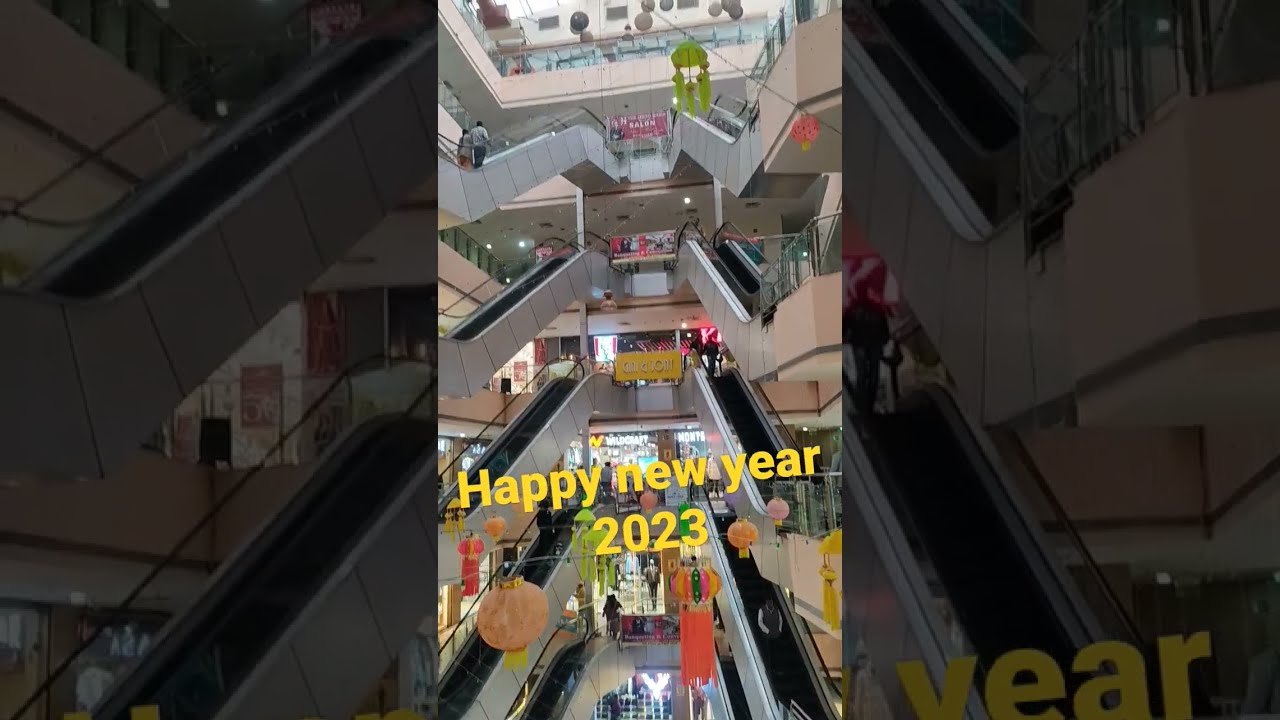The image is a vertically oriented photo taken inside a multi-story shopping mall, prominently featuring five or six levels of interconnected floors. The central section, framed by dimmed, zoomed-in segments of the same image on the left and right, shows an interior view looking towards a back wall adorned with storefronts and various decorations, including colorful paper lanterns. The mall's architectural layout includes beige and gray walls, with escalators positioned on both sides, facilitating movement between the levels. People can be seen milling about on the lower floors. The open courtyard design allows visibility across the different stories, complete with railings and escalators forming a visually striking pattern. Yellow text at the bottom of the central image reads "Happy New Year 2023."